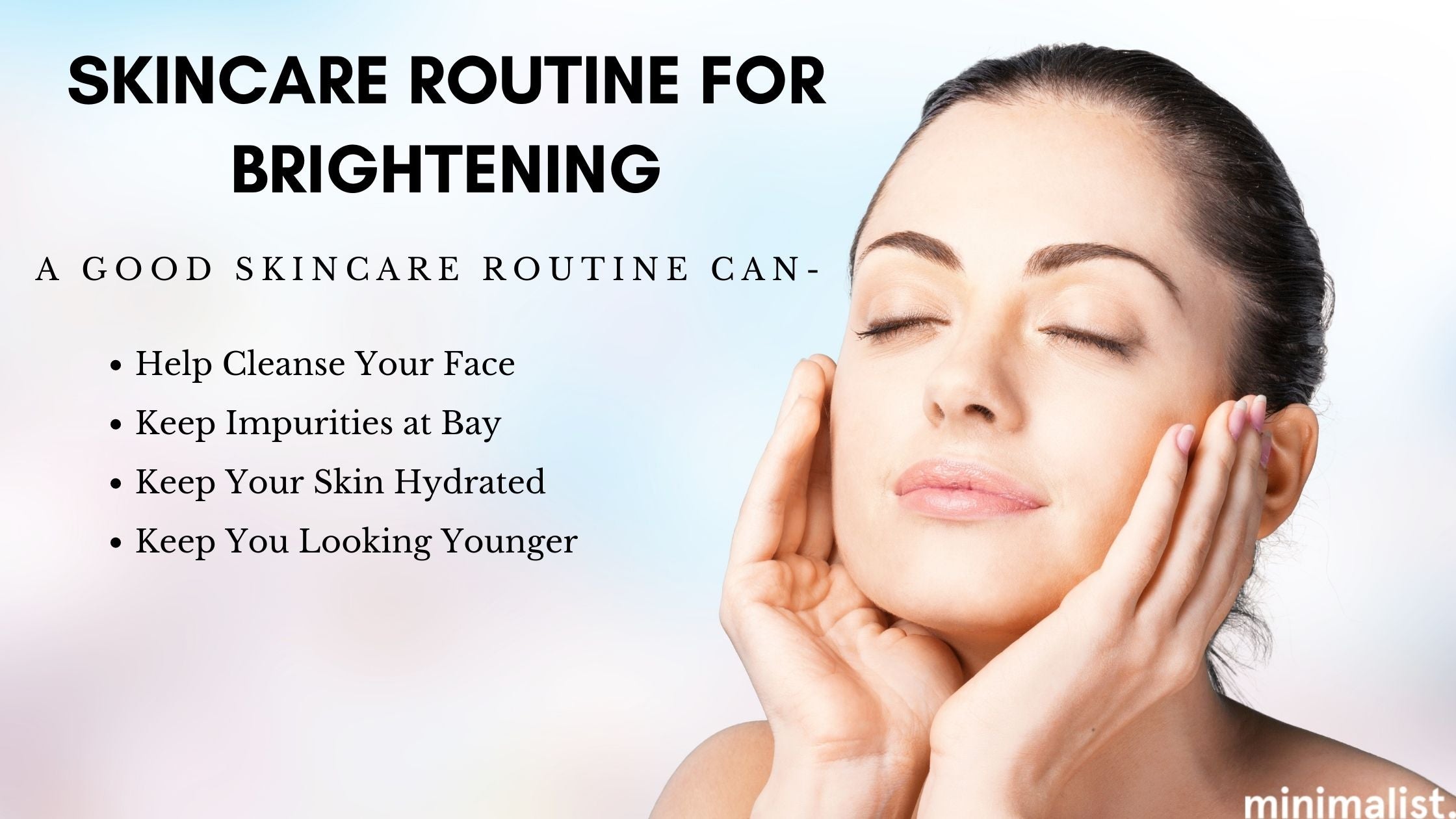The image is a full-color, digitally enhanced horizontal rectangle without a border, primarily featuring light shades of blue, white, purple, and pink in the background. In the lower right-hand corner, white lowercase letters spell out "minimalist." Dominating the upper left-hand corner are bold black letters proclaiming, "skin care routine for brightening." Below this title, smaller black text reads, "A good skin care routine can:" followed by bullet points listing the benefits: help cleanse your face, keep impurities at bay, keep your skin hydrated, and keep you looking younger. The central figure is a young Caucasian woman with her eyes closed, her hands gracefully positioned on either side of her face as she applies a skincare product. She has brown hair, defined eyelashes, and pouty lips. Her serene expression and healthy, radiant skin epitomize the advantages of an effective skincare regimen.